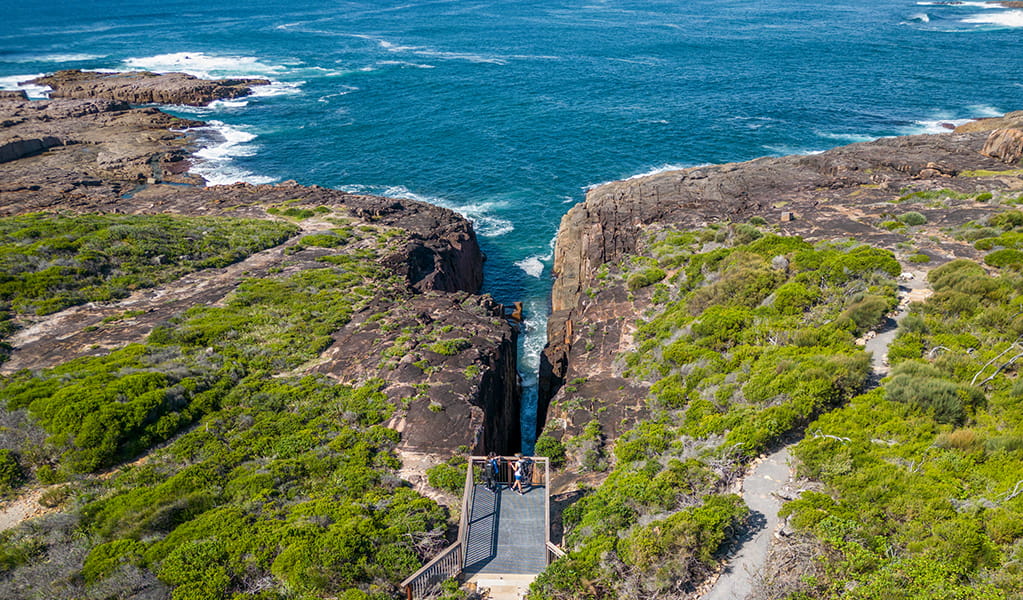This aerial image captures a dramatic landform that has been split into two expansive masses of dark brown and gray rock, forming a striking crevice that houses a narrow waterway. This waterway, seen in vivid blue, stretches from the lower part of the image, meandering through the rocky divide, and leads out to a larger lake, which occupies the top of the image and extends beyond the frame. The lower middle section of the image features an observation deck with a blue bottom, serving as a vantage point over this scenic split. Two people can be seen standing on the deck, highlighting its scale. 

Flanking the waterway, the rocky terrain on both sides exhibits a sparse distribution of light green bushy vegetation, with more greenery concentrated toward the middle and lower parts of the image. The left side of the split showcases more gray rock interspersed with green bushes. Towards the upper left, the rocky coast meets the lake, where white waves are visibly splashing against the stones. The right side of the image features green trees and a cleared path that leads towards a stone cliff, also displaying some wave activity on the lake. This juxtaposition of rugged rock formations, verdant vegetation, and tranquil blue water creates a captivating natural landscape.